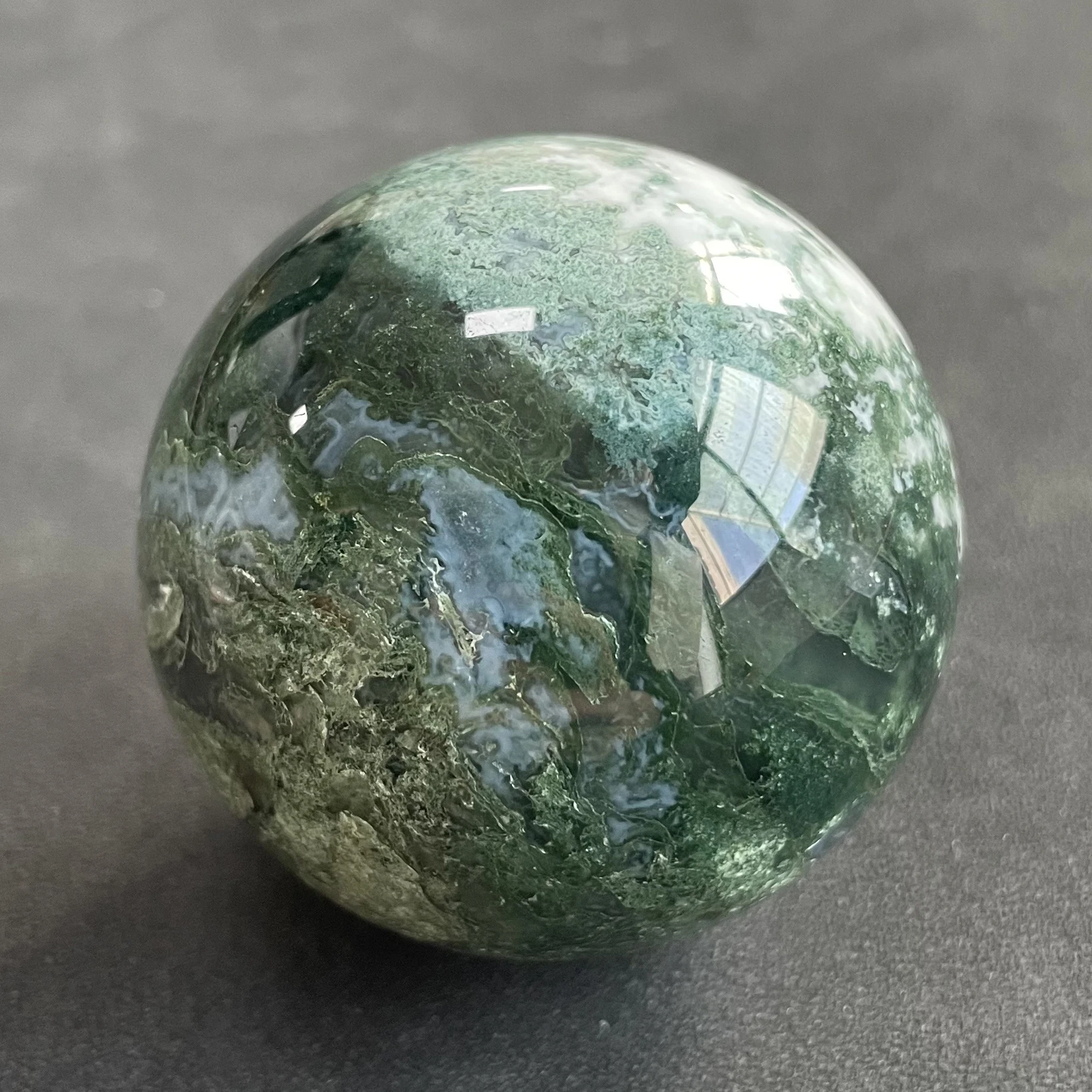This photograph showcases a perfectly polished, shiny sphere resting on a textured, light gray surface. The image is slightly angled, capturing a side view while looking slightly down on the sphere. The sphere appears to be made from a blend of materials, possibly resembling melted silver on its lower left side, transitioning to various shades of milky green and dark green. This intricate, glassy sphere, which could be a gemstone or a geological substance like quartz, exhibits significant shine and reflection. Notably, reflections of rectangular windows can be seen on the upper right side of the sphere. The background is blurred towards the top, with the detailed gray surface visible in the lower half, all framed within a roughly square image.